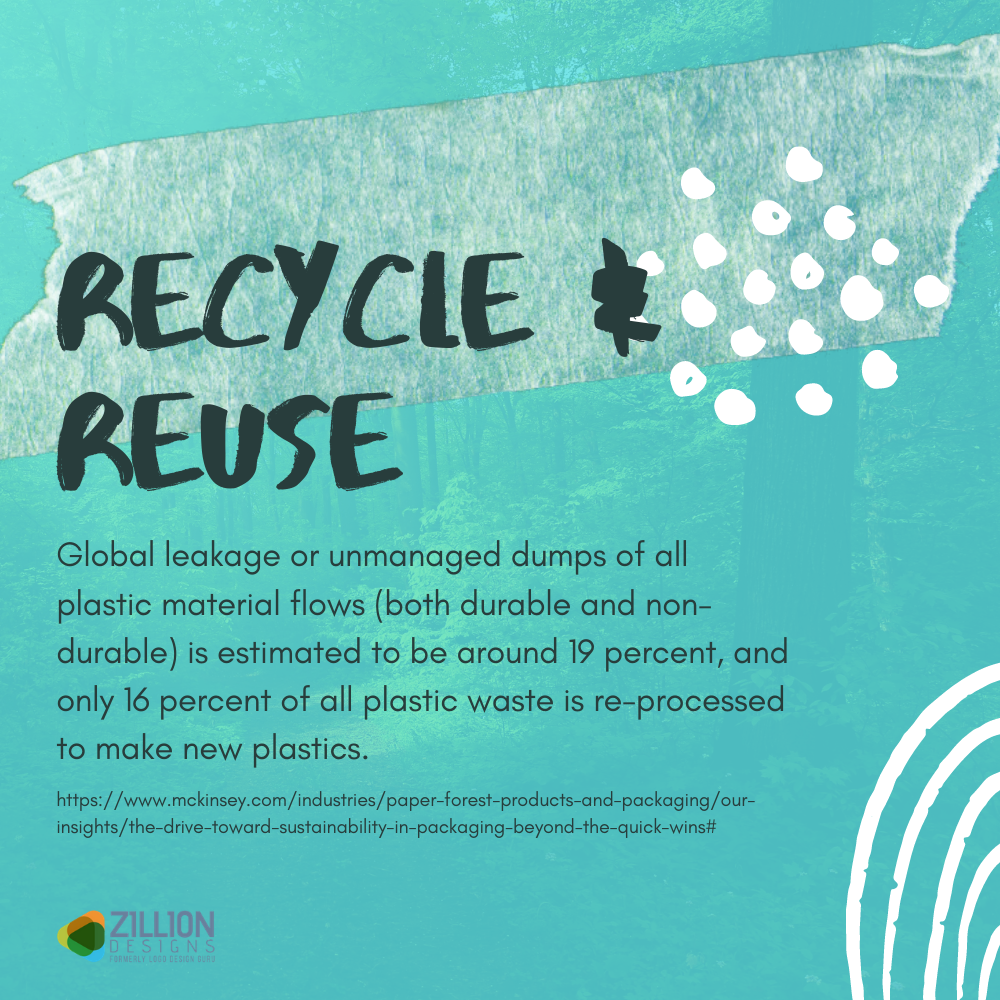This poster, designed by Zillion Designs, features a square layout with a light turquoise blue background, complemented by a mottled pattern of darker green hues resembling bushes and trees. At the top of the poster, there is a faded piece of tape adorned with small white decorative dots. Centered on this tape are two prominent lines of black text reading "Recycle" on the first line and "Reuse" on the second. Below this headline, additional black text provides important information: "Global leakage or unmanaged dumps of all plastic material flows, both durable and non-durable, is estimated to be around 19%, and only 16% of all plastic waste is reprocessed to make new plastics." In the lower right-hand corner, there are a series of delicate curved white lines for added decoration. The lower left-hand corner features the Zillion Designs logo in green, white, and orange. The poster also includes a URL for further information: "https://www.mckinsey.com/industries/paper-forest-products-and-packaging/our-insights/the-drive-towards-sustainability-in-packaging-beyond-the-quick-wins". The overall intent of the poster is to promote the significant message of recycling and reusing plastics.